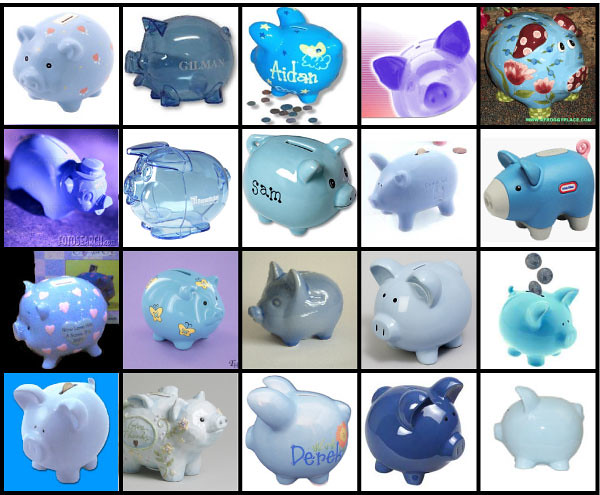This photo showcases a meticulously arranged grid of twenty piggy banks, distributed across five columns and four rows. Each square in the grid contains a uniquely designed piggy bank, predominantly of porcelain with a few made from see-through plastic. The color palette ranges from light blue, dark blue, aqua blue to white, with various intricate patterns. 

Notable designs include a piggy bank painted with blue flowers, another adorned with butterflies and stars, and one bearing the name "Aiden" in white. In the top-left corner, there is a light blue piggy bank with pink hearts, followed by a transparent dark blue piggy bank, a dark blue one with white butterflies and stars, and a light purple one with prominent purple ears in the center row. 

The second row from the top features three basic blue piggy banks on the left and another blue one surrounded by a few scattered coins. A distinctive block-shaped dark blue piggy bank with a gray nose and feet is also present. In the third row, a dark gray piggy bank sits beside a blue one with pink hearts and another with yellow butterflies. Additional blue variations, including sky blue and light blue, are also present.

The bottom row includes a light blue piggy bank with detailed etchings and another labeled "Derek" in dark blue. The lower right corner showcases another light blue piggy bank. Throughout the image, these piggy banks display unique designs and colors, highlighted against a backdrop dotted with a few coins, adding to the charm of the collection.